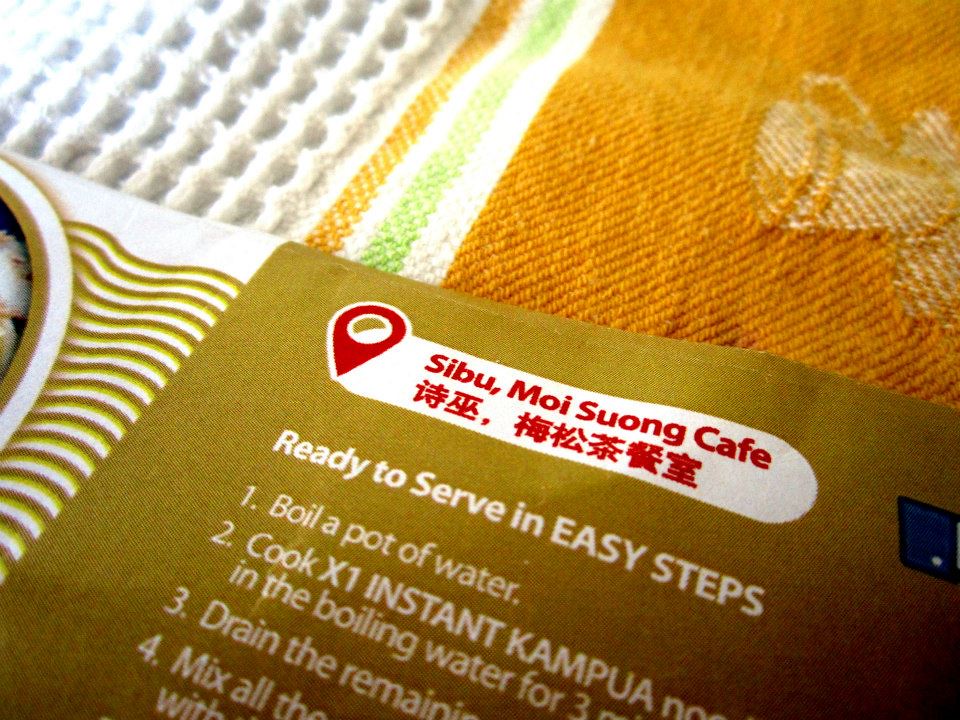The photograph captures a vibrant and colorful scene, featuring half of a meal label alongside a piece of fabric that appears to be either a placemat or a napkin. The fabric is bright and lively, displaying colors such as bright white, orange, light orange, yellow, and green with a waffle-knit pattern and stripes of orange and green. Additionally, there is an embroidered or printed image of a small teacup or coffee cup with a saucer in shades of orange and light orange.

The label, originating from a cafe named "Sibu Moi Suwon Cafe," contains partial directions for preparing an instant meal. It reads, "Ready to serve in easy steps," followed by the steps: "1. Boil a pot of water. 2. Cook x1 instant kampua in the boiling water for..." and then it is cut off. The text continues with, "3. Drain the remaining..." and is cut off, ending with the instruction, "4. Mix all...," but the remainder of the directions is also not visible. This incomplete label is juxtaposed against the colorful fabric, leaving a visually dynamic and intriguing composition.